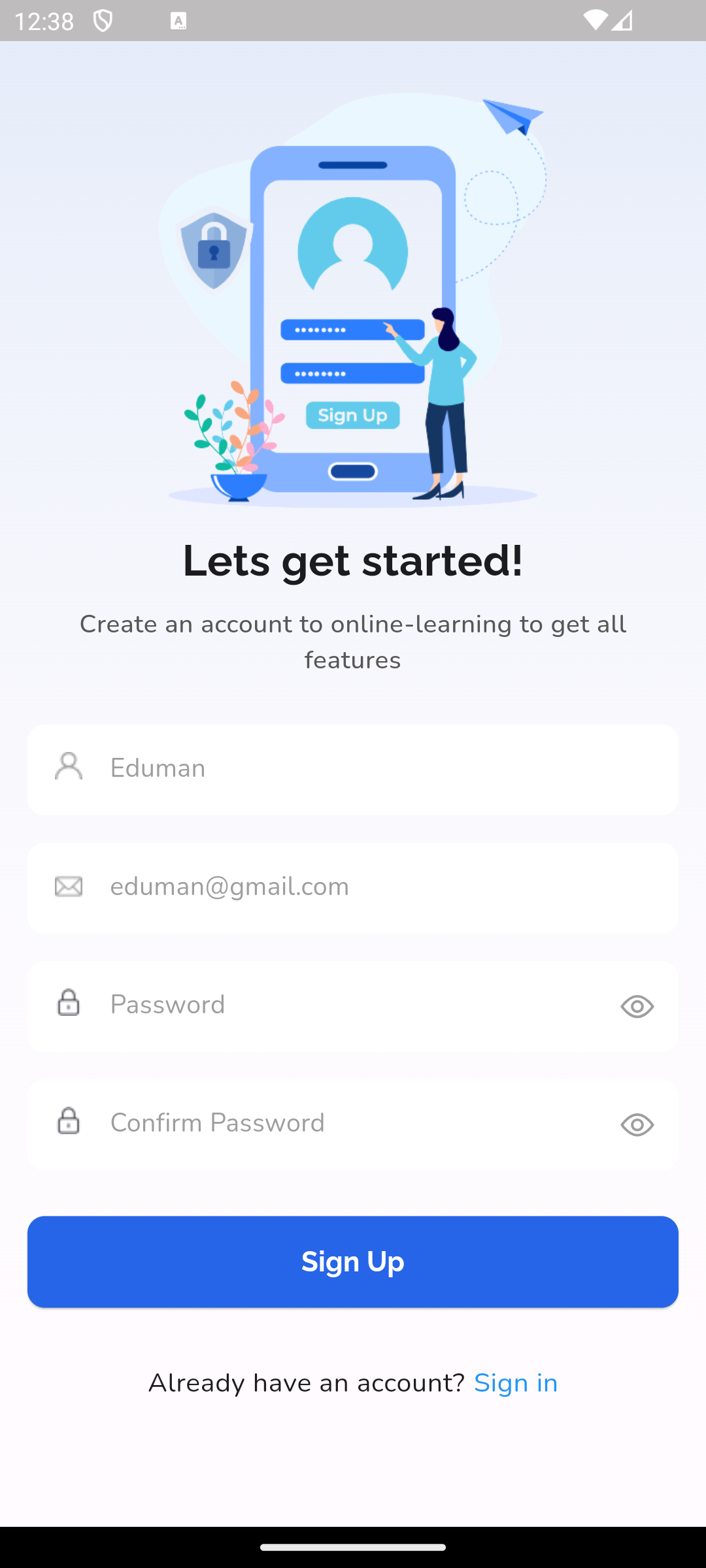This image is a screenshot from a smartphone display. The background color transitions from a very light blue at the top to white towards the bottom. At the top border, which is gray, the time '12:38' is displayed in white on the left.

The top third of the screen features a simple graphic within the light blue section. This graphic depicts a giant smartphone with a woman standing in front of it, about half the height of the smartphone. The main portion of the screen within the giant smartphone's display has a white background.

The graphic inside the smartphone screen includes a small symbol at the top representing an account, depicted as a round circle on top of a semi-circle. Below this symbol, there are two oblong blue boxes. Further down, there is a light sky-blue box with the text "Sign Up" in white font.

Directly beneath the graphic, in black headline text, it says "Let's Get Started." Below that, in gray font, it reads "Create an account to online learning to get all the features." There are subsequent fields for the user to input their name, email, password, and confirm password.

At the bottom of the screen, there is a blue rectangle with rounded corners that contains the text "Sign Up" in white font.